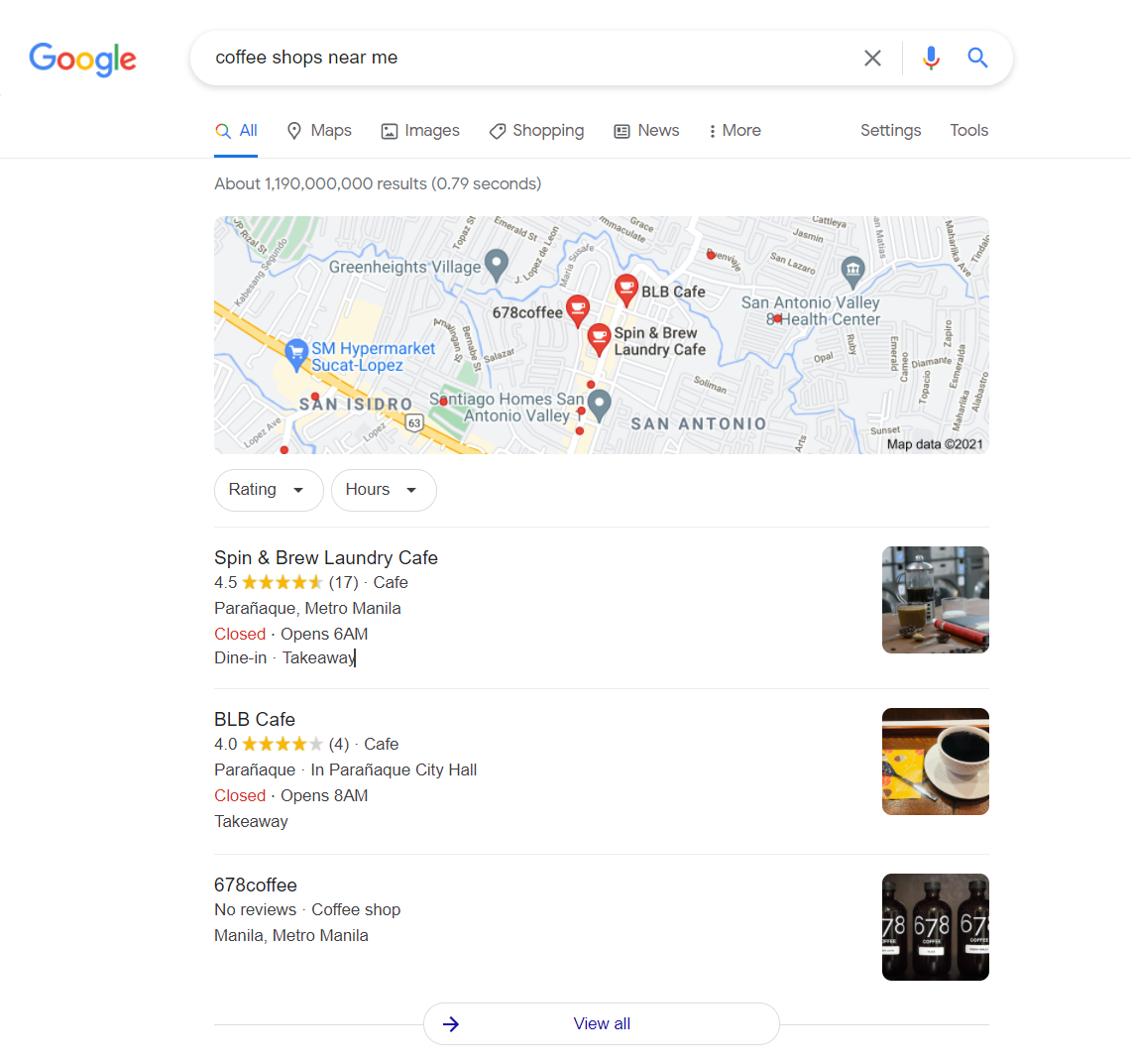The image depicts a Google search results page with the familiar Google logo in the top left corner, displaying the iconic blue, yellow, red, and green colors. Next to the logo, there is a white search bar containing the query "coffee shops near me" in black text. Below the search bar, there are various tabs: "All," "Maps," "Images," "Shopping," "News," "More," "Settings," and "Tools." The "All" tab is currently selected, showing approximately 1,190,000 results found in 0.79 seconds.

There are three coffee shops pinned on the map, indicated with red markers. The first listing is "Spin & Brew Laundry Cafe," rated 4.5 stars based on 17 reviews. It is located in Parañaque, Metro Manila, and is noted to open at 6 AM with options for dine-in and takeaway. Adjacent to this listing is a photo of the establishment.

Following a gray divider, the second coffee shop listed is "BLB Cafe," rated 4.0 stars from four reviews. It is also situated in Parañaque, Metro Manila, specifically near the City Hall, and it opens at 8 AM offering takeaway services. A photo accompanies this listing as well.

The final listing, "678 Coffee," does not have any reviews yet. It is categorized as a coffee shop located in Manila, Metro Manila, and is accompanied by a photograph.

The background of the entire page is white, providing a clean and simple visual layout.